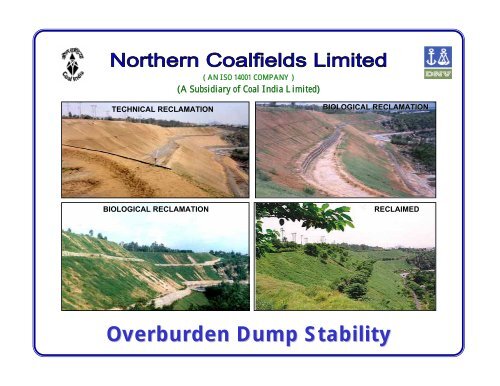This advertisement for Northern Coalfields Limited (a subsidiary of Coal India Limited) features a sequence of four images showcasing different stages of land reclamation. The top left image, labeled "Technical Reclamation," depicts a dry, yellowish landscape primarily covered in dirt. Adjacent to it on the top right, labeled "Biological Reclamation," shows the same area with initial patches of greenery starting to appear. The bottom left image, also termed "Biological Reclamation," presents a further developed landscape with significantly more green vegetation covering most of the brown dirt. Finally, the bottom right image, titled "Reclaimed," displays a lush, verdant scene teeming with grass, bushes, and trees, indicating the completion of the reclamation process. Beneath these images, the text "Overburden Dump Stability" is written in blue, all set against a white background with a blue border along the sides.